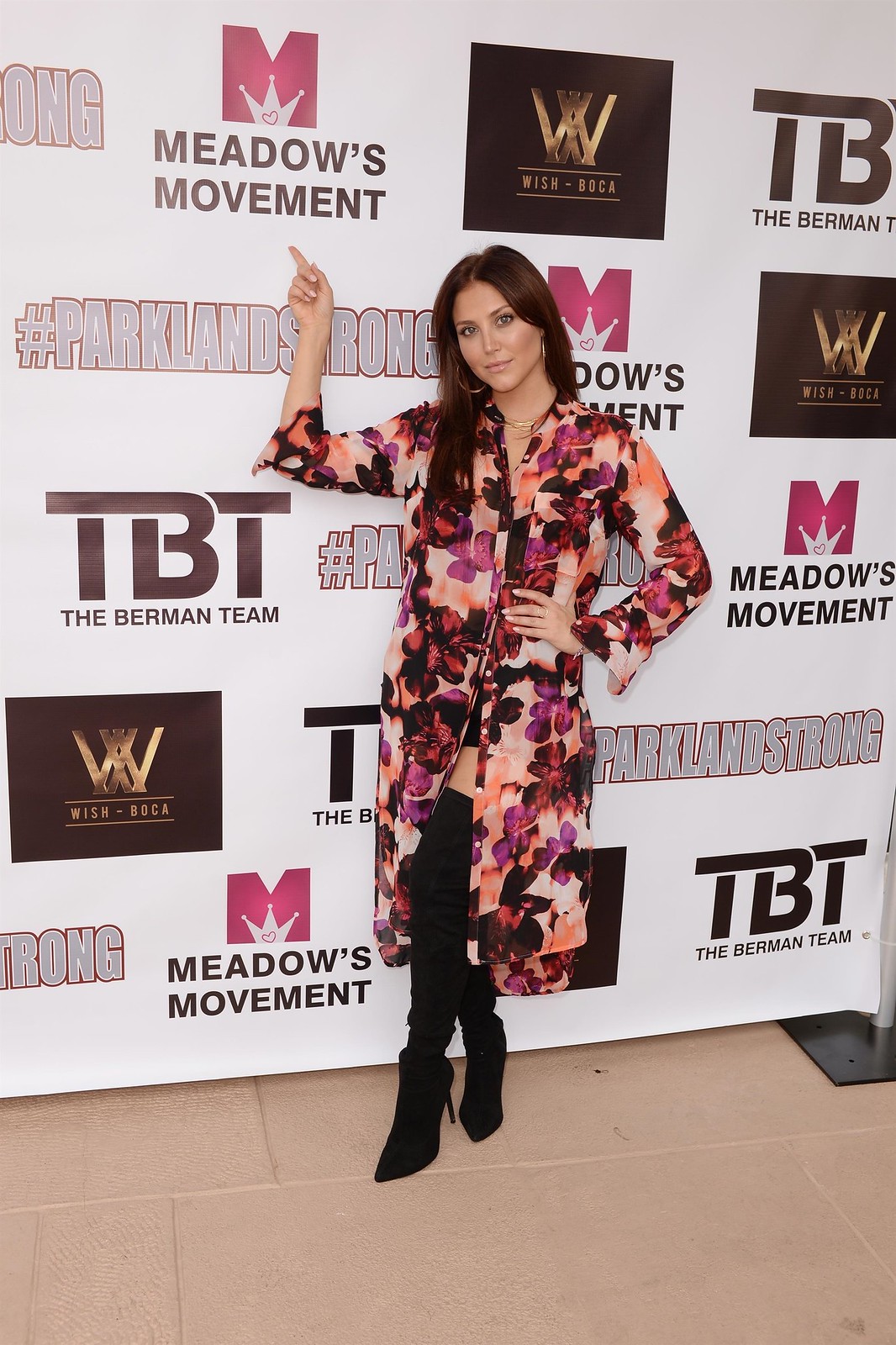The image captures a stylish event reminiscent of a fashion show backdrop. At the center stands an attractive woman with brown hair, adorned in large hoop earrings. She exudes confidence in a chic, long, floral-patterned coat that flows open to reveal her elegantly positioned leg in thigh-high, sexy black boots. The floral coat, an artful blend of purple, red, black, and cream elements, drapes superbly below her knees and hints at her navel through its open front, complemented by unbuttoned sleeves.

She directs attention to a sign on the white background with light brown lettering that reads "Meadows Moment," prominently featuring a red ‘M’ topped with a regal crown. Surrounding her are various logos on a white wall banner, including 'TBT, The Berman Team' in brown, 'Wish Boca' denoted by a gold 'W' in a dark brown square, and multiple #ParklandStrong hashtags. The entire scene is set against a cream-colored tile floor, with the overall palette harmonizing pink, cream, black, and white tones, underscoring both sophistication and elegance at the event.